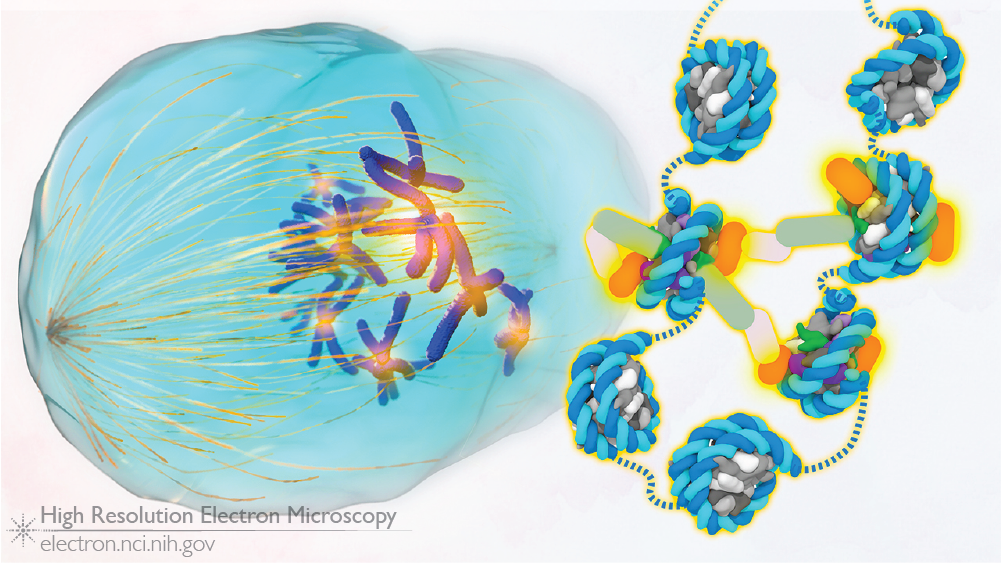This highly detailed, colored image resembles an animated drawing, set against a white background. On the bottom left corner, the image is annotated with "High Resolution Electron Microscopy" in gray, underlined text, followed by a URL, "electron.nci.nih.gov." Dominating the left side is a large, wavy blue structure, threaded with white and yellowish-orange lines that extend in multiple directions. Adjacent to this, on the right side, are clusters of cylindrical shapes in varying shades of blue, some intertwined with larger green cylindrical pieces. These clusters, connected by small green dots, spiral upwards and out of the frame. The interconnected structure continues downward, merging into a dense ball of mixed blue, light green, gray, and white cylindrical components. The intricate detail and coloration highlight the complex, viral-like entities, accompanied by DNA or molecular structures intricately woven together.